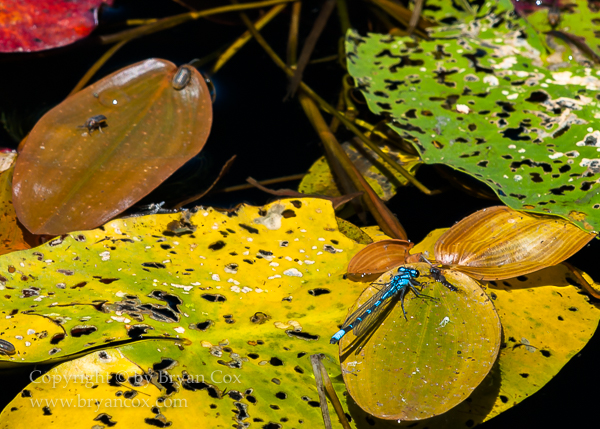This vibrant photograph, taken by Brian Cox, showcases a variety of wet leaves floating in dark water, creating a striking contrast. Dominated by different shades and textures, the image features a mix of green, yellow-green, and reddish-brown leaves, some of which have prominent black holes or freckles on them. The upper right corner reveals a brownish-green leaf hosting two small beetle-like bugs. In the lower half of the picture, a larger yellowish-green leaf, marked by black spots, overlaps slightly with other leaves and displays a striking blue dragonfly with black accents. This blue dragonfly, with its elongated body and several legs, shares the space with another insect nearby. The scene is set against a black background, amplifying the vivid colors and details, with the photographer's name and website, www.briancox.com, visibly noted at the bottom.